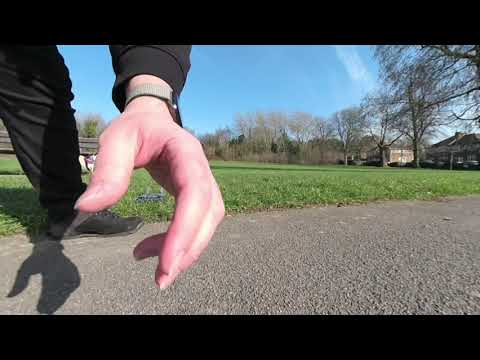The photo captures an outdoor scene centered around a camera placed on a grey asphalt or concrete path. The left side of the image is dominated by a man's left hand, extending from the top towards the center, casting a distinct shadow on the ground. The man, who appears to be wearing a black shirt, black pants, and black shoes, also sports a wristwatch with a beige or light-colored band, resembling an Apple Watch. Visible near the bottom of the image is part of his leg. The background reveals a scenic, peaceful setting with a lush green grassland leading up to rows of trees, under a bright blue sky dotted with occasional white clouds. Behind the man stands a wooden bench, and beyond the trees, several buildings of brick construction—potentially houses, dorms, or office buildings—enhance the rural or serene atmosphere of the scene.